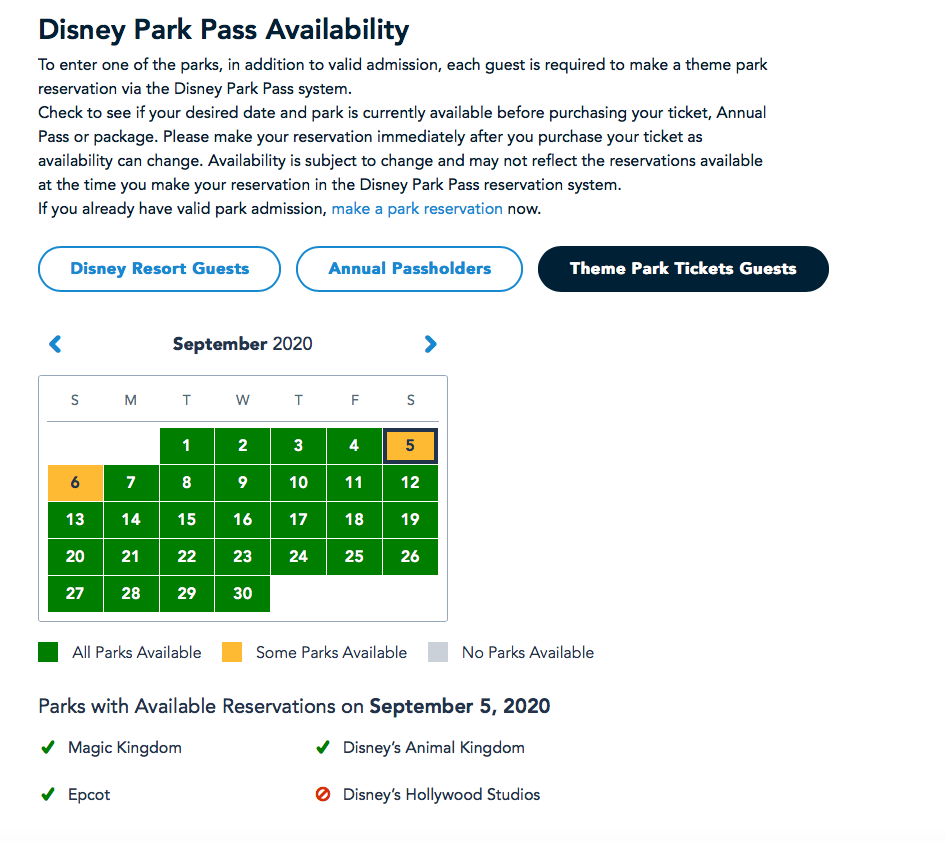A computer printout displays information regarding Disney Park Pass Availability for September 2020. The calendar highlights that, for most days of the month, all parks are available except for the 5th and 6th of September, which are noted as Labor Day weekend. Specifically, on the 5th of September, Disney's Hollywood Studios is the only park that is not available for reservations, while Magic Kingdom, Epcot, and Disney's Animal Kingdom remain open for bookings.

The printout also includes an important notice informing guests that, in addition to a valid admission ticket, a theme park reservation via the Disney Park Pass system is required to enter any park. Users are advised to check the availability of their desired date and park before purchasing a ticket, annual pass, or package. Prompt reservation is encouraged immediately after ticket purchase, as availability can fluctuate. The notice emphasizes that reservation availability is subject to change and may not reflect real-time status in the Disney Park Pass system. Guests who have already secured valid park admission are urged to make their reservations promptly.